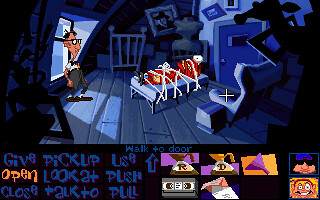The image appears to be a screenshot from a video game, characterized by a classic adventure game interface. At the bottom of the screen, there is a black border featuring several options in blue text, arranged in three rows of three words each: "give", "open", "close", "pick up", "look at", "talk to", "use", "push", and "pull". Notably, the word "open" is highlighted in orange, indicating it is currently selected. Above this border, there is an arrow pointing upwards towards the phrase "walk to door", accompanied by various colored icons—purple, orange, black, brown, white, red, and more—likely representing character options or possible interactions.

In the main play screen, a man stands in the foreground wearing thick-rimmed glasses, a white shirt tucked into high-waisted gray pants, white socks, and dark shoes, presenting a stereotypically nerdy appearance. He is positioned in front of a window, looking at another figure who is completely dressed in white, including a white mask that barely reveals colored eyes. This figure, who also wears a red outfit beneath white ropes that bind him, appears to be tied to a flat surface, possibly a bed. Behind this scene, a blue door with a window at its top can be seen, leading to what looks like a storage area filled with boxes and miscellaneous objects.